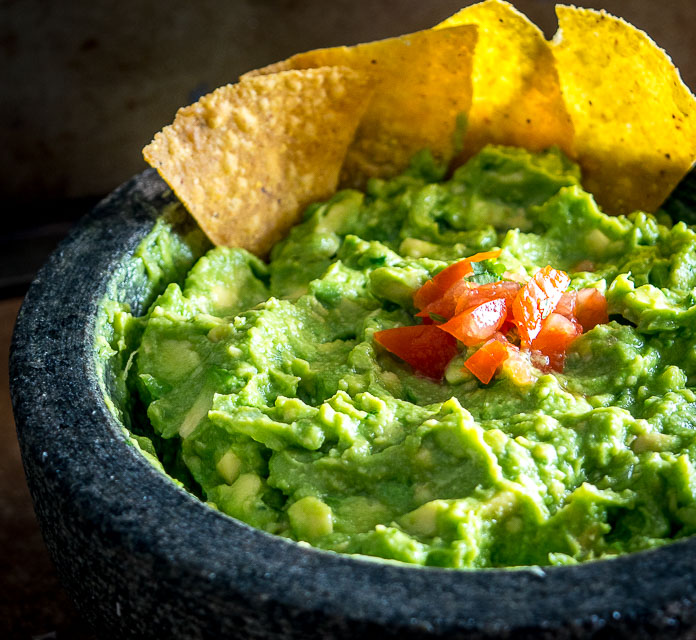The image features a close-up of a traditional molcajete, a stone mortar used for grinding ingredients, originating from a specific region in Mexico. The molcajete, colored a dark gray, holds freshly crushed avocado, forming a creamy guacamole. Atop the guacamole are pieces of either diced tomato or red pepper, adding a vibrant touch of red. Tortilla chips are strategically placed upright around the molcajete, ready to be dipped into the flavorful sauce. The scene beautifully showcases the authentic preparation and presentation of a classic Mexican dish.